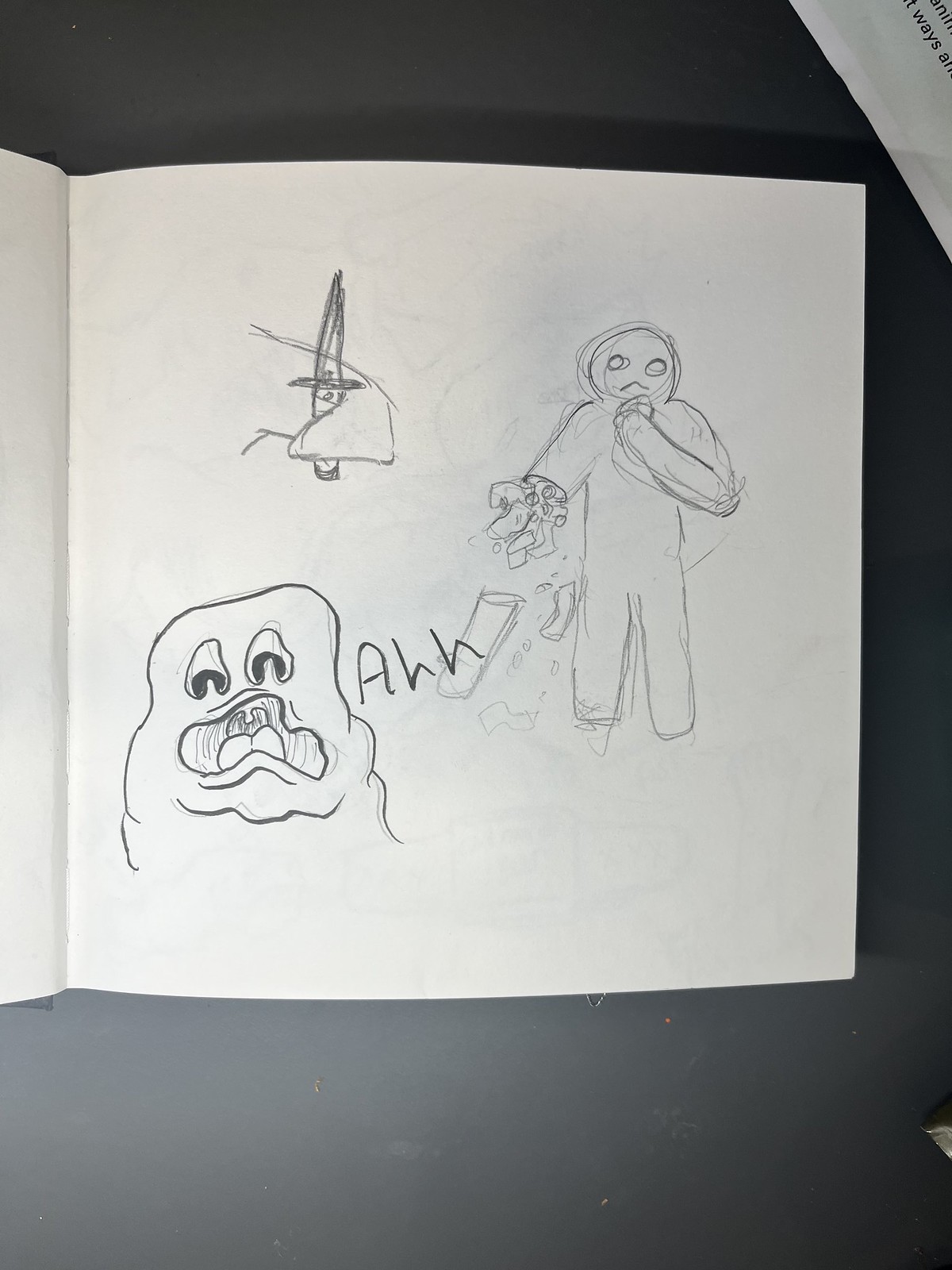This monochromatic pencil drawing depicts a spectral figure reminiscent of Slimer from the Ghostbusters franchise. The ghostly character is centrally positioned and is vocalizing an "AHH," inscribed within the image. The artwork is on a plain sheet of white paper, which has been folded to suggest it might form a booklet. The background consists of a slate-grey tabletop.

In the upper right corner of the composition, there's a partially visible inscription that seems to read something about "weighs", though the text is indistinct and likely part of another document. On the right side of the ghostly figure is a gingerbread man with a severely damaged right arm, appearing as if it has been bitten off and mangled. To the upper left of the gingerbread man, an ominous hand holding a switchblade knife can be seen, adding a sense of impending peril to the scene.

The overall use of pencil on paper, paired with the specific elements and their placement, creates a striking and eerie visual narrative.